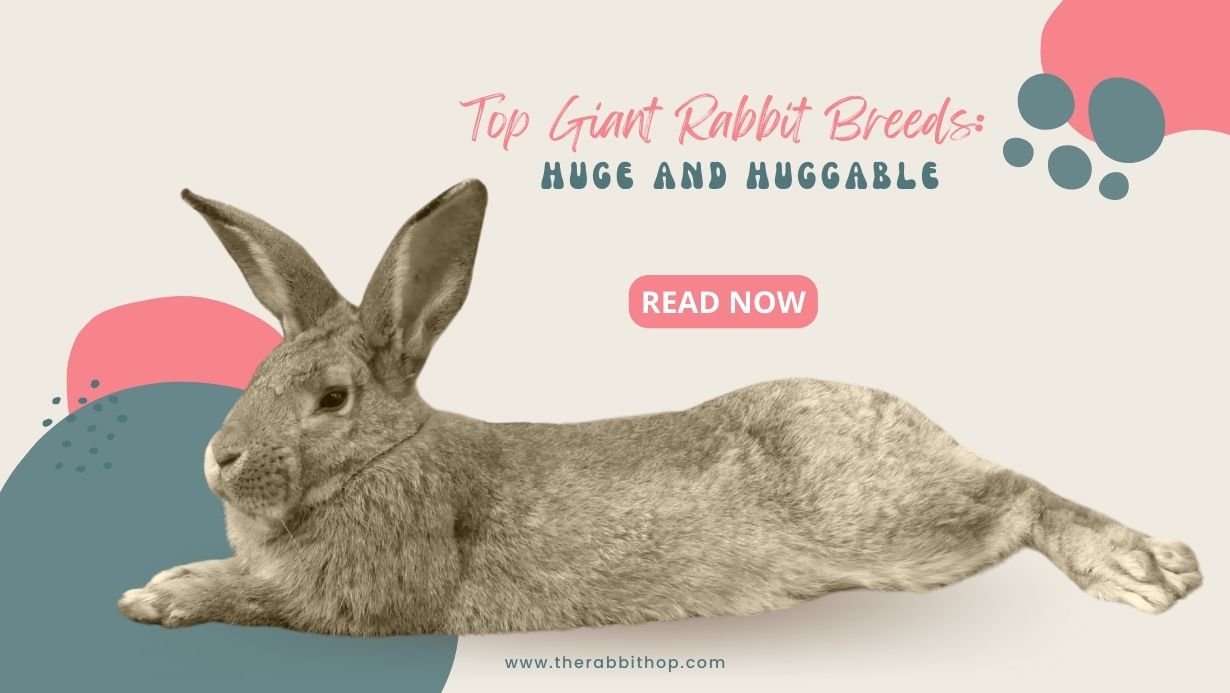At the bottom of a webpage from "therabbitshop.com," there is an advertisement featuring a light tan background with abstract splotches of muted pink and teal colors. Dominating the image is a photograph of a bunny lying down with its feet behind it and ears pointed straight up. The bunny has an off-brown taupe and cream-colored coat, with lighter hues in its ears and darker shades on its back, along with black eyes.

Above the bunny, in large, bold text, are the words "Top Giant Rabbit Breeds" in pink, and "Huge and Huggable" in a muted teal color. Below these descriptions, there is a pink button with white font that says "Read Now." The website’s name "therabbitshop.com", in teal, is positioned simply at the bottom of the advertisement. 

The ad also features a decorative design element on the left side, consisting of scattered teal dots, numbering about fifteen in total. This setup appears to be part of a larger website, possibly placed as an advertisement in a rabbit enthusiast forum.